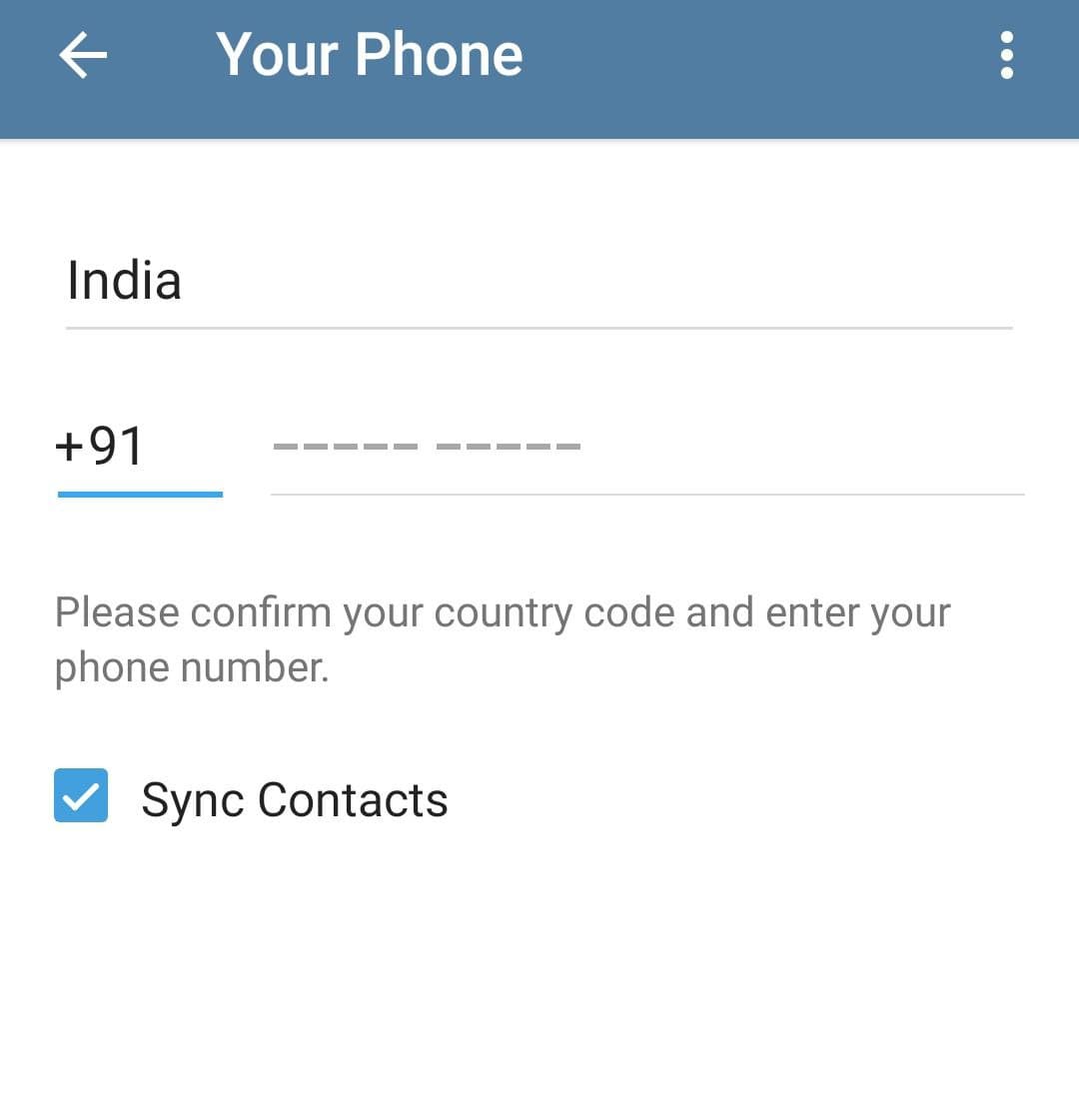This image is a screenshot taken from a phone. The top of the screen features a light blue horizontal band stretching from left to right. On the left side of this band, there is a white arrow pointing to the left. To the right of the arrow, the words "Your Phone" are displayed in white text. At the far right end of the blue band, three vertical white dots are aligned flush with the edge.

Below this band, the background is white. Just underneath, there is a thin gray line stretching across the screen, with the word "India" typed in dark letters on it. Below this, the next line is underlined in teal, where in black letters, the code "+91" is typed, followed by a space. To the right of this, there is another thin gray underline with gray placeholders above it, indicating spaces for digits of a phone number, arranged as five dashes followed by another five dashes.

Further down, gray text reads: "Please confirm your country code and enter your phone number." At the bottom of the screen, there is a medium blue rectangular button with a white check mark within it. To the right of this button, "Sync Contacts" is displayed in black text.